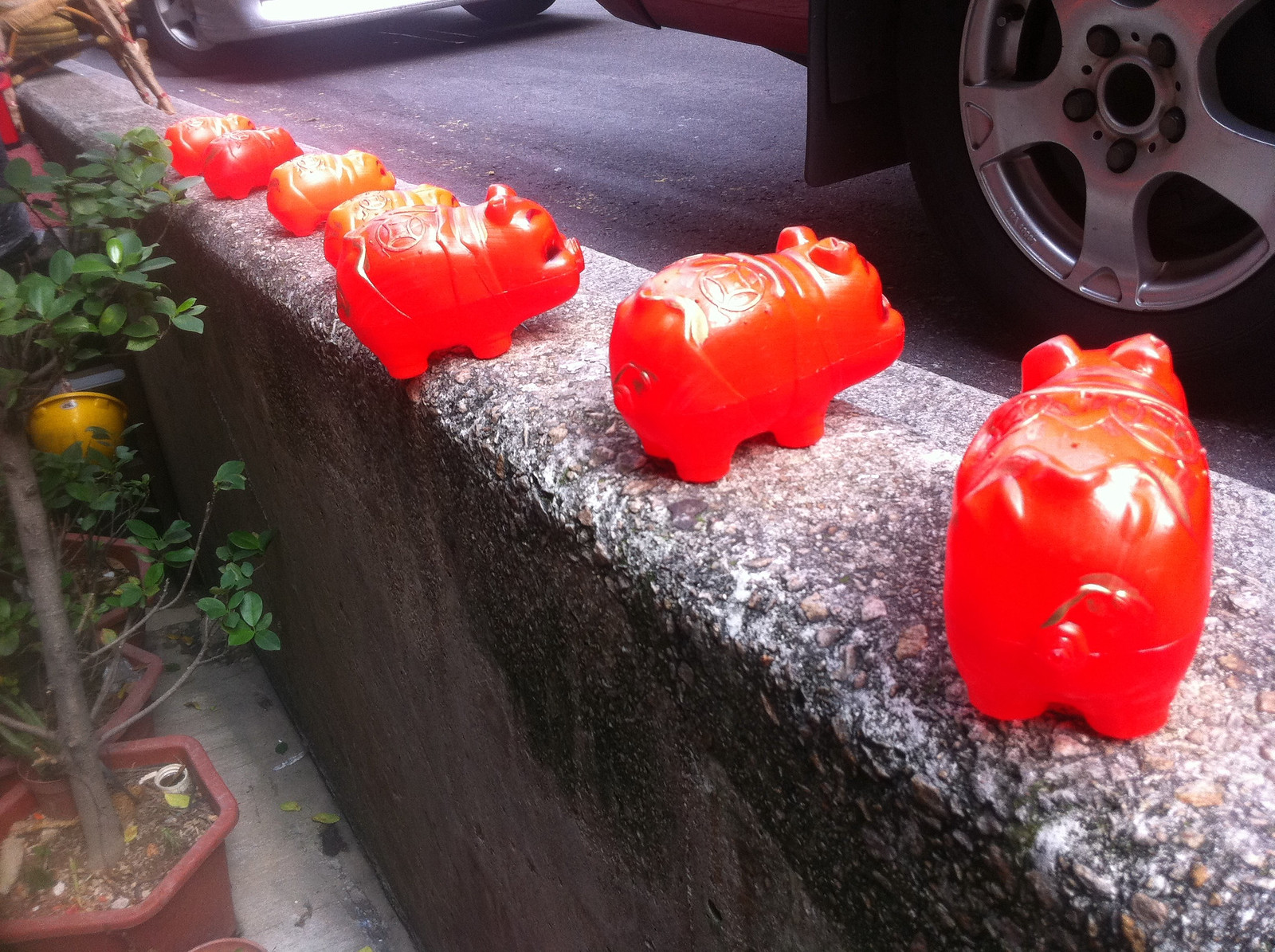This image captures a line of seven decorative red pig figurines, reminiscent of plastic piggy banks but without any coin slots, neatly arranged on a brick or stone retaining wall. They are all uniformly facing outwards towards a street. Although the street itself is cut off, the direction is indicated by the partial view of two parked cars – one white and one red – visible through glimpses of their tires and bumpers. Behind the pig figurines, on the inner side of the wall, lies a residential patio area with various potted plants and a yellow bowl, suggesting a cozy, outdoor domestic setting. The scene is brightly lit, indicating that the photograph was taken during the day.